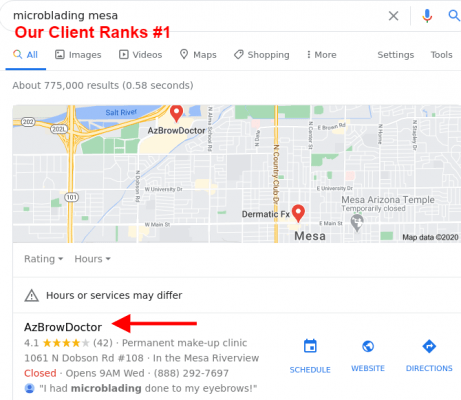The screenshot displays a Google search results page for "microblading Mesa." At the top, in blue text, is the word "All" with a blue underline indicating the selected tab. Adjacent to it in gray text are other options: "Images," "Videos," "Maps," "Shopping," and "More." To the right, the "Settings" and "Tools" options are visible.

Below this row, there is a narrow segment of a map highlighting parts of Mesa, Arizona, with location pins marked for "AZ Brow Doctor" and "Dramatic FX." The search results show AZ Brow Doctor's details: a permanent makeup clinic located at 1061 North Dobson Road, Suite 108, within the Mesa Riverview area. It has a rating of 4.1 stars and is closed at the moment, with an opening time of 9 a.m. on Wednesday. The contact number provided is 888-292-7697. A red arrow points to this listing, emphasizing it, and there's an included quote from a customer stating, "I had microblading done to my eyebrows."